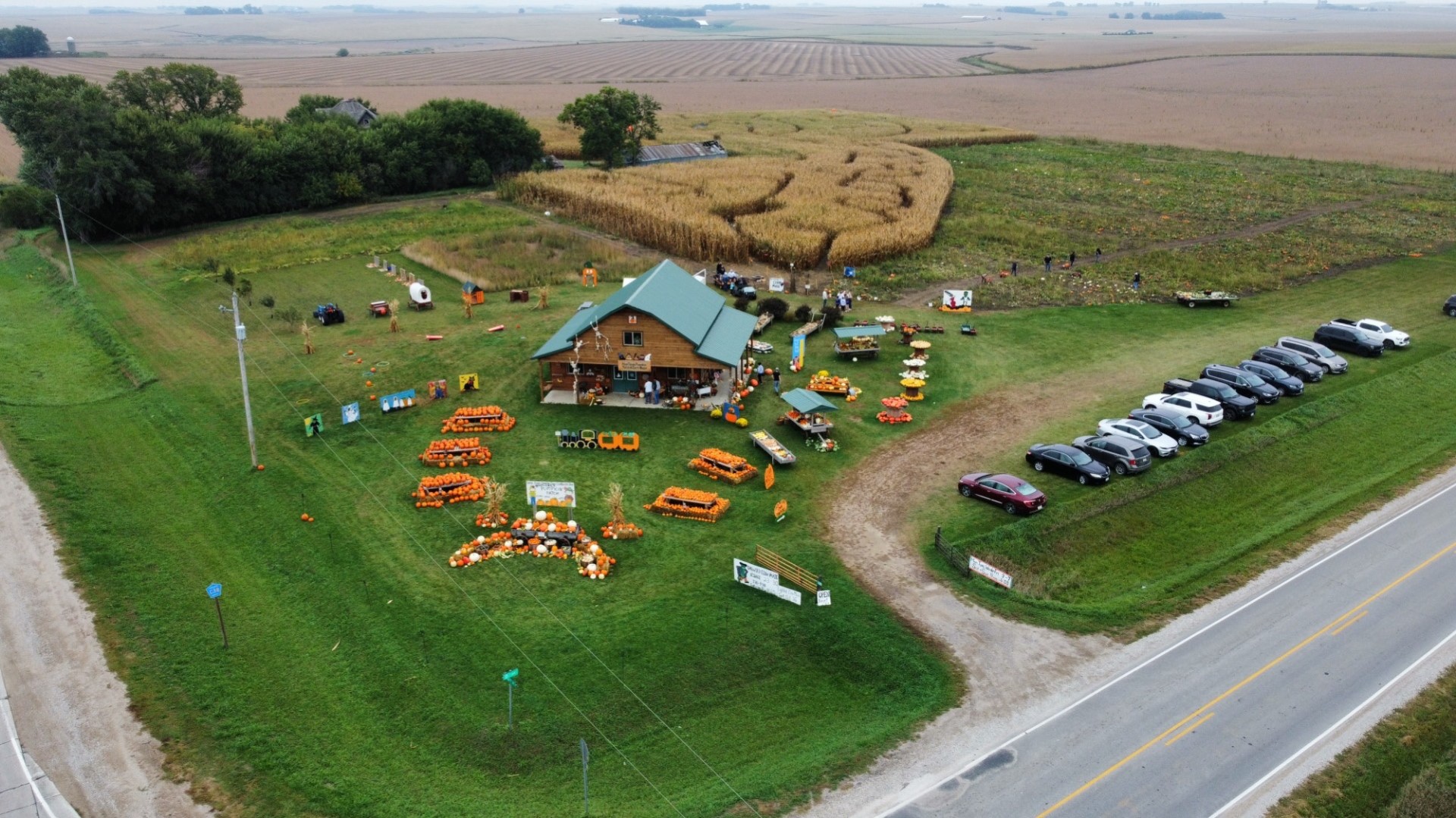This aerial photograph captures a bustling farm scene on a bright, sunny day. The image showcases a farm with verdant green grass, juxtaposed with fields of brown and yellow, indicative of both living and dead crops. In the upper right corner, there is a wheat field, while the bottom left harbors a grassy dirt parking lot occupied by at least a dozen cars. The farm is bordered by a copse of trees on the top left and lined with a road featuring yellow and white lines along the bottom edge. 

Centrally, there is a prominent farmhouse-like building with a green pointed roof, displaying stacks and columns of pumpkins, implying a festive, possibly autumnal, atmosphere. Picnic tables around the building are similarly decorated with squashes or pumpkins, accompanied by farm-related outdoor attractions such as wagons filled with fruits. There are signs indicating perhaps market stalls or informational posts. 

In the background, there is a sprawling field marked with high, uncut corn forming pathways suggestive of a corn maze, hinting at seasonal activities on the farm. People can be seen scattered across the area, engaging with the attractions and exploring the grounds. Power lines run along the front of the property, which provides an additional, faintly modern touch to this otherwise pastoral scene.